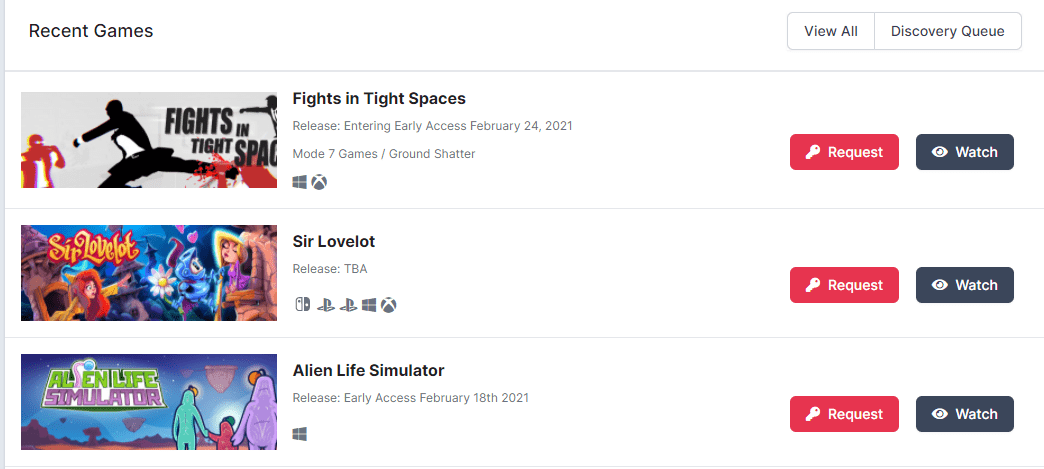A detailed and cleaned-up caption for the described image could be:

---

The image appears to be a screenshot from a gaming app or digital storefront, likely the Google Play Store or Apple App Store. The banner at the top of the screen features the header "Recent Games" on the left. On the right side of the banner, there are two rectangular buttons: "View All" and "Discovery Queue."

Below the banner, three game options are displayed prominently:

1. **Fights in Tight Spaces**: An image in red, white, and black depicts intense fighting scenes. The details accompanying the image indicate that the game entered Early Access on February 24, 2021. The developers are Mode 7 Games and Ground Shatter. Red "Request" and black "Watch" buttons are available beneath the game title.
   
2. **Sir Love Lot**: This game features a colorful, cartoon-style image with various women, flowers, and hearts. The release date is listed as TBA (To Be Announced). Red "Request" and black "Watch" buttons are available for this title as well.
   
3. **Alien Life Simulator**: The image shows a person holding hands with a small alien, with a larger alien standing to their right. The game details indicate that it entered Early Access on February 18, 2021. The "Alien Life Simulator" title is displayed above the image, and it also has red "Request" and black "Watch" buttons.